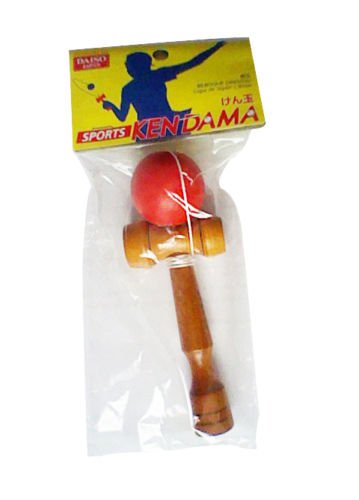The photograph showcases a kendama toy, often referred to as the ball and cup toy, still encased in its original packaging. The toy is displayed on a flat surface, yet the white background of the photograph gives it an ethereal appearance, as if it were suspended in a white void. The kendama is packaged in a clear plastic bag, sealed at the top with a vibrant yellow tag. This tag features a blue outline of a person playing with the kendama and has a hole punched for display hanging.

Prominently, the top left corner of the yellow tag bears a red rectangle with white text that reads "Daiso," indicating the Japanese manufacturer. The tag also features another red rectangle in the bottom left corner, labeled "Sports" in white text. Adjacent to this, in red text with a white outline, is the word "Ken Dama." The toy itself is composed of a wooden hammer-like handle with a rope attaching a rubber ball to it, showcasing its traditional design.